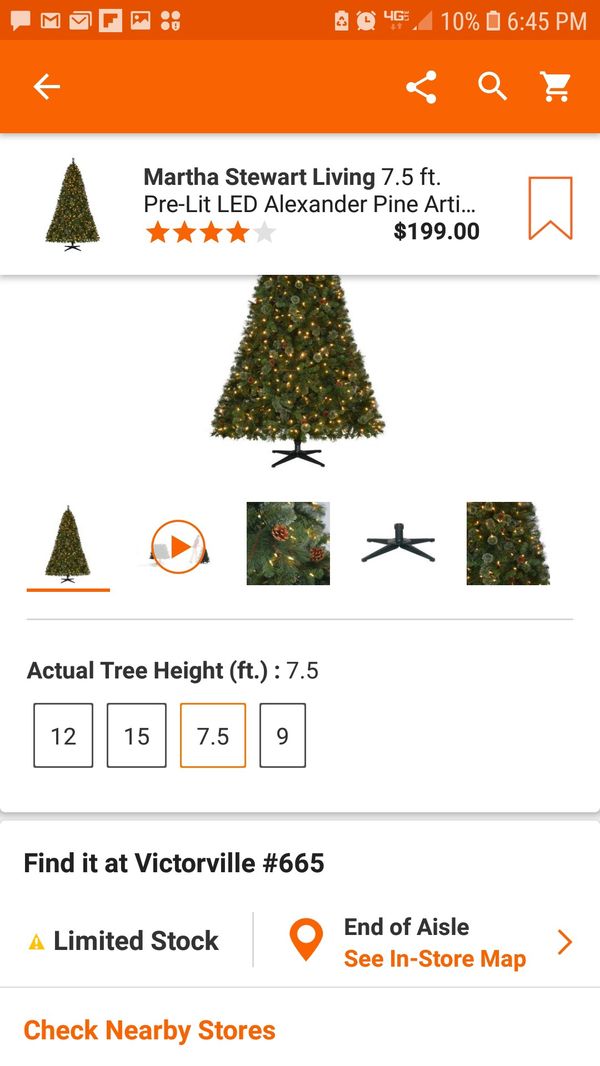The image displays a mobile view of a website, presumably from Home Depot, given the orange hue of some of the text on the screen. The screen shows a product listing for a pre-lit artificial Christmas tree, specifically the "Martha Stewart Living 7.5 feet Pre-Lit LED Alexander Pine," priced at $199.00. The item has a four-star rating. Details include a selection of videos and images showcasing the tree's illuminated appearance.

In the upper left corner of the screen, typical mobile interface icons are visible: a messaging app icon, Gmail icon, data signal icon, a 10% battery life indicator, and the current time displayed as 6:45 PM. Navigation elements like a back arrow, share button, search icon, and a shopping cart icon are also present.

The listing specifies that the tree’s actual height is 7.5 feet. Availability is limited, noted by the text "Find it at Victor L 665 Limited Stock End of Aisle See in Store Map," and it also provides an option to check stock in nearby stores.